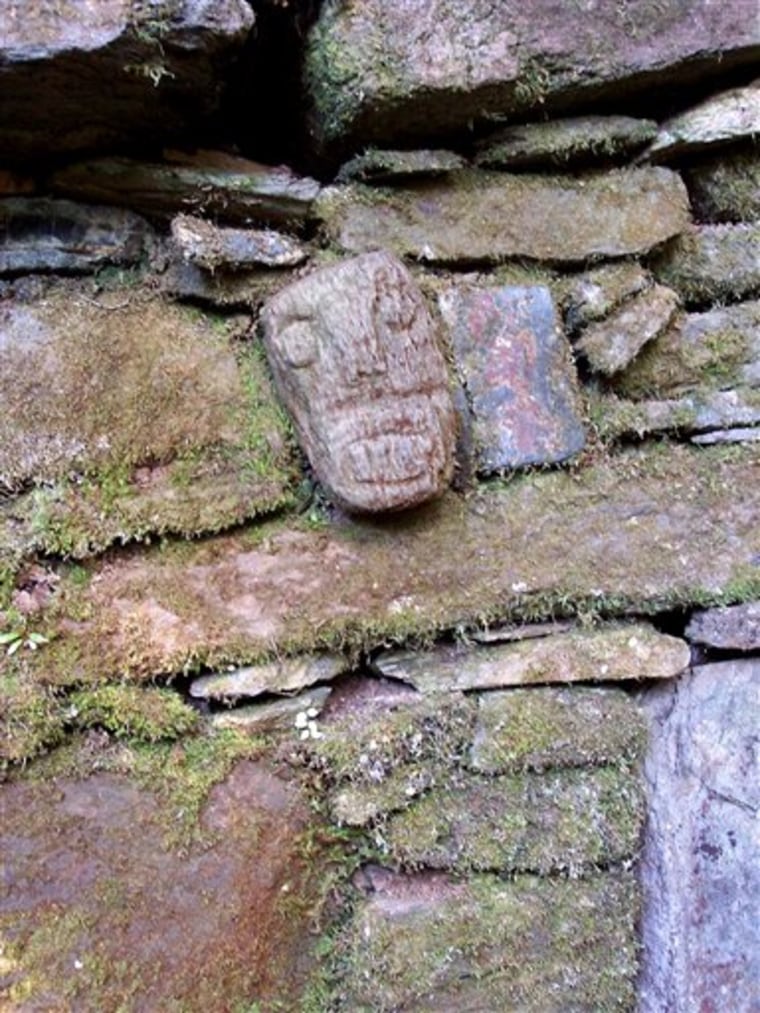In this detailed outdoor photograph, we see a densely packed stone wall featuring a multitude of rocks, some of which are layered and adorned with naturally occurring grass, moss, and lichen. Prominently positioned in the center of the image is a distinctive ancient-looking gray stone, meticulously carved to resemble a face with two eyes, a long nose, and a mouth. This carved face is surrounded by a variety of other stones, each with its own unique characteristics: to the left, a moss-covered rock; below, a spherical-shaped stone; and to the right, a purple and blue rock. The bottom right corner features a smooth blue and gray rock. The environmental conditions suggest a damp area, possibly with a water source, as the rocks appear wet and some are muddied. Above the carved stone face, additional gray rocks are visible, further adding to the earthy, textured composition. The photograph captures the intricate details of the stone arrangement and the natural elements thriving among them.